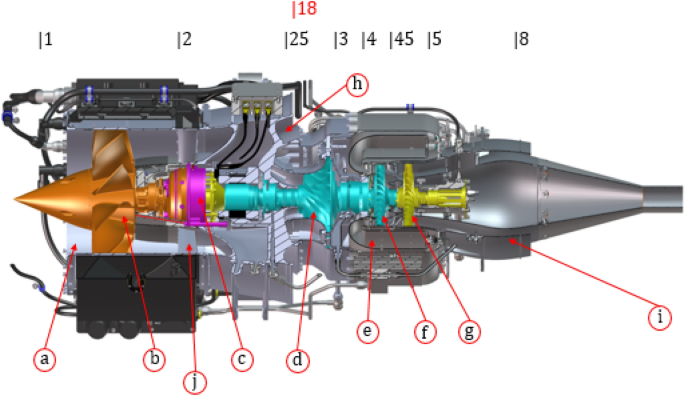This is a detailed technical diagram of what appears to be a cross-sectional view of a mechanical engine or weapon, depicted in a landscape-oriented, color illustration style. The diagram features a variety of gears and internal components, differentiated by distinct colors: orange, pink, blue, yellow, and gray. Along the top of the image, there is a row of bracketed numbers including 1, 2, 25, 3, 4, 45, 5, and 8.

Red circular callouts with black text letters A, B, J, C, D, E, F, G, H, and I are used to label various parts of the mechanism, with red arrows indicating the specific areas of interest. On the left-hand side, labels A and B point to an orange section that is protruding outward. In the center, labels J and C highlight a pink ring connecting the orange part to a turquoise or aqua section denoted by labels D and E. The right side features labels F, G, and I, which point to a gray section towards the rear of the engine.

The diagram includes a blowout label system, with detailed red arrows leading to red outlined circles, each labeled with a letter that corresponds to different parts of the internal mechanism. Adding to the complexity, the left side of the illustration shows a bullet-shaped copper-colored projectile pointing leftwards, indicating its relation to the overall mechanism. Overall, this intricate and vibrant technical drawing serves as a likely excerpt from a textbook or technical manual.